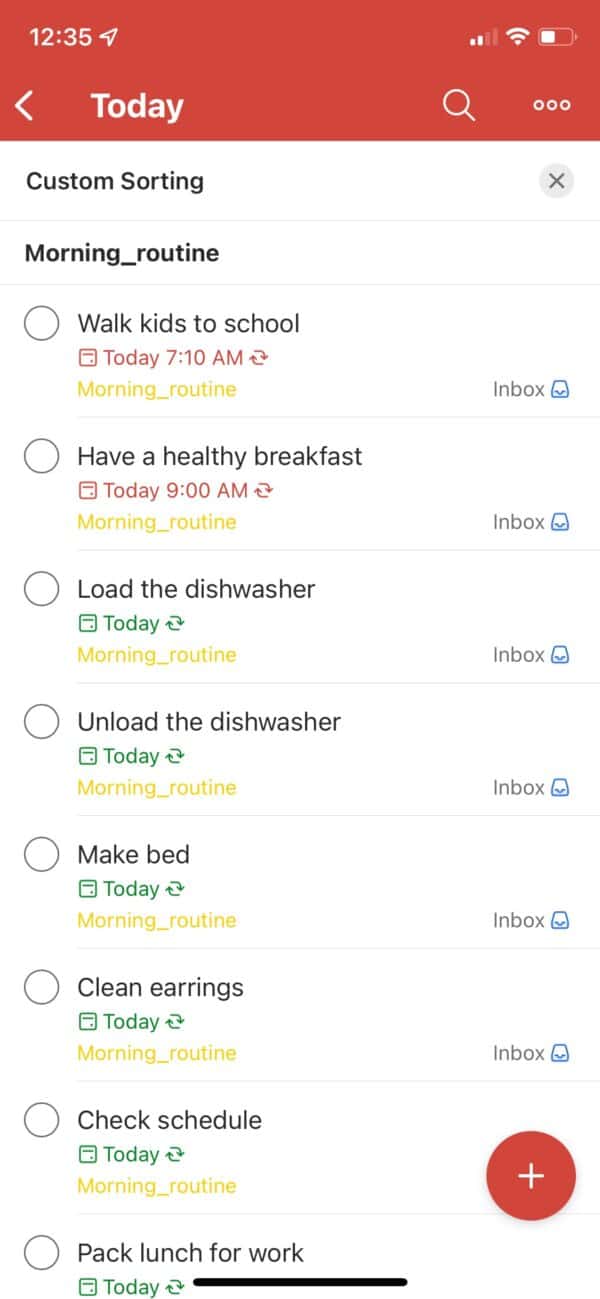Here is a detailed and cleaned-up caption for the image:

---

This image is a screenshot from an iPhone, displaying the "Reminders" app. The screenshot shows that the time is 12:35 PM, and the phone is connected to Wi-Fi with approximately 50% battery remaining. The banner at the top is an orangey-red color and features a white left-arrow labeled "Today," a magnifying glass icon, and three horizontal dots located towards the right.

Below the banner, the screen displays a white background with black text that reads "Custom Sorting" with an "X" icon opposite to it. The primary focus of the screenshot is a list titled "morning_routine," which comprises several tasks each marked by checkable dots. The tasks are as follows:

1. Walk kids to school today at 7:10 AM – highlighted in yellow under the "morning_routine" category.
2. Have a healthy breakfast today at 9:00 AM.
3. Load the dishwasher today.
4. Unload the dishwasher today.
5. Make bed today.
6. Clean earrings today.
7. Check schedule today.
8. Pack lunch for work today.

Each task also has an option to move it to the inbox, denoted by an inbox icon on the right. At the bottom right corner of the screen is a reddish-orange circle with a white plus sign, likely used to add new tasks to the routine.

---